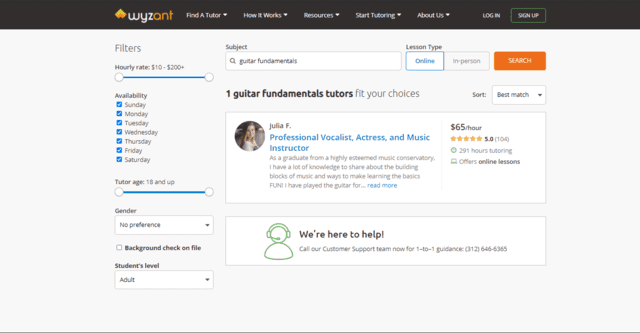This image is a horizontally-oriented screenshot from the website of a company named "Wyzant," a platform for finding tutors. At the top of the image, a thin black banner spans the width of the page, prominently featuring the company's name "Wyzant" with the letters "W-Y-Z" in white font and "A-N-T" in orange font. To the left of the company's name is their logo, which is a combination of yellow and orange tones.

Adjacent to the company name, several drop-down sections in small white text are displayed, including "Find a Tutor," "How It Works," "Resources," "Start Tutoring," and "About Us." Additionally, the banner includes options for "Login" and "Sign-Up," with the sign-up box highlighted with a green outline.

On the left side of the page, there is a vertical column designed for filtering search results. This column includes a slider to adjust the hourly rate, checkboxes to select availability by day (Sunday through Saturday), and a slider bar for the tutor’s age. Further options include a drop-down box for selecting the tutor's gender, a checkbox for background checks, and another drop-down box to specify the student's level.

At the top of the page, there is a search bar that allows users to specify the subject and lesson type. In this instance, "Online" has been selected for the lesson type. To the right of the search bar, there is an orange search button.

Below this, the search results are displayed, indicating that "One Guitar Fundamentals Tutor" fits the specified criteria. The highlighted tutor is Julia F., a professional vocalist, actress, and music instructor. Positioned to the left of her information is her profile picture. Julia F. charges $65 per hour and has a 5-star rating. Beneath her information, an icon of a person with a microphone signifies customer support, accompanied by the text, "We're here to help."